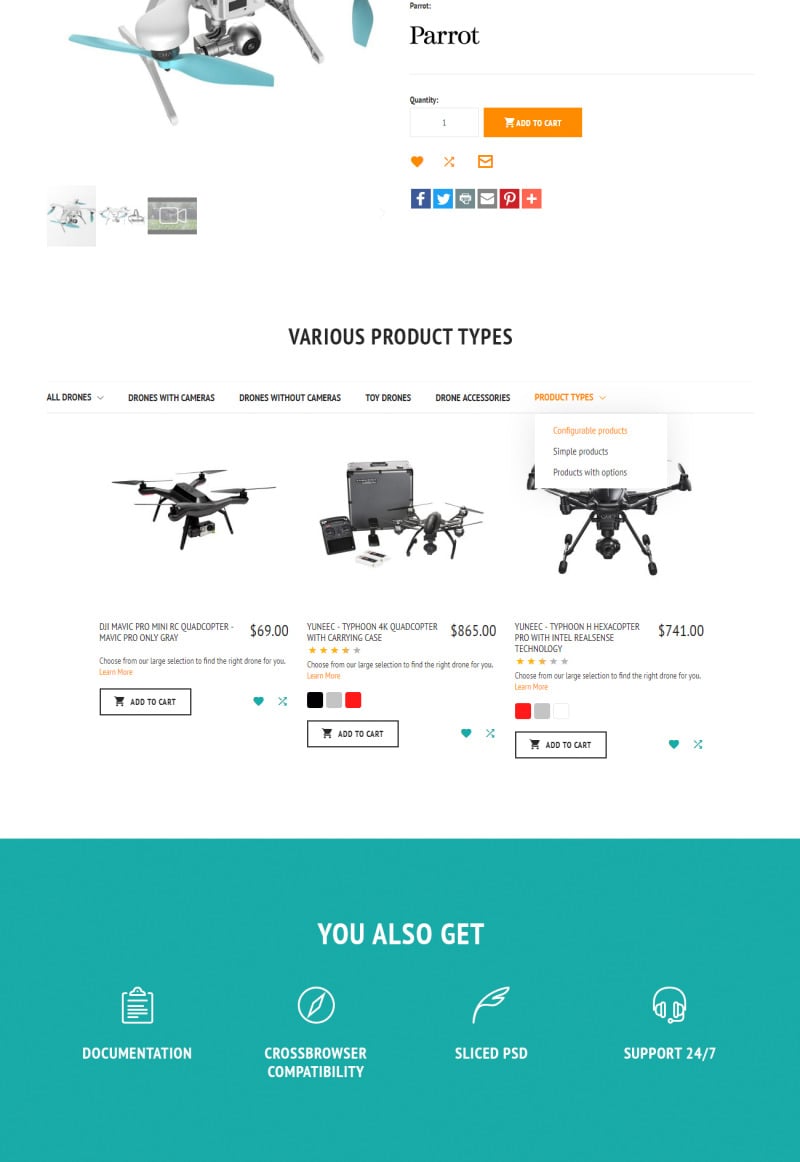In the image, there is a section displaying a variety of drones and related products. On the left, there is text showing a quantity selector with "1" as the default value and an "Add to Cart" button situated to the right of the text.

The image features an assortment of drone categories and product types, including:

- **All Drones**
- **Drones with Cameras**
- **Drones without Cameras**
- **Toy Drones**
- **Drone Accessories**

Under the "Product Types" dropdown menu, options such as "Configurable Products," "Simple Products," and "Products with Options" are available.

Several specific drone models are highlighted:

- **DJI Mavic Pro**
- **Mini RC Quadcopter**
- **Yuneec Typhoon 4K Quadcopter with Carrying Case**
- **Yuneec Typhoon H Hexacopter Pro with Intel RealSense Technology**

Each drone model is depicted with its corresponding features, capturing the diversity and advanced technology available in the current drone market.